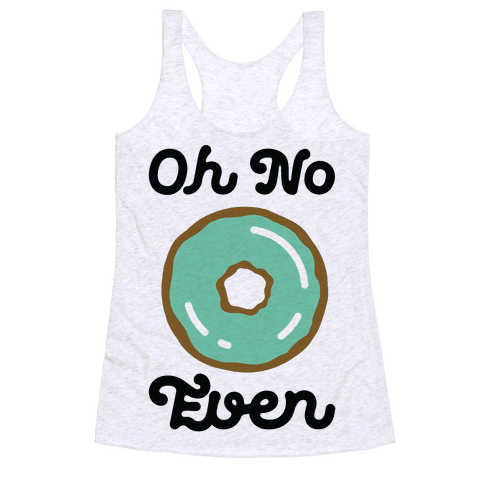The image features a sleeveless racerback tank top displayed against a white background. The tank top is made of a very light gray, heathered fabric, almost appearing whitish. Prominently displayed on the front, the tank top features playful, large, black cursive text. At the top, it reads "oh no," while at the bottom, it says "even." These phrases bracket a central graphic of a donut. The donut has a brown outline with frosting in a tealish-green color, adorned with white lines and a dark outline in the center, mimicking a sprinkled effect. The overall design seems to evoke a humorous and whimsical vibe, suitable for a female audience.